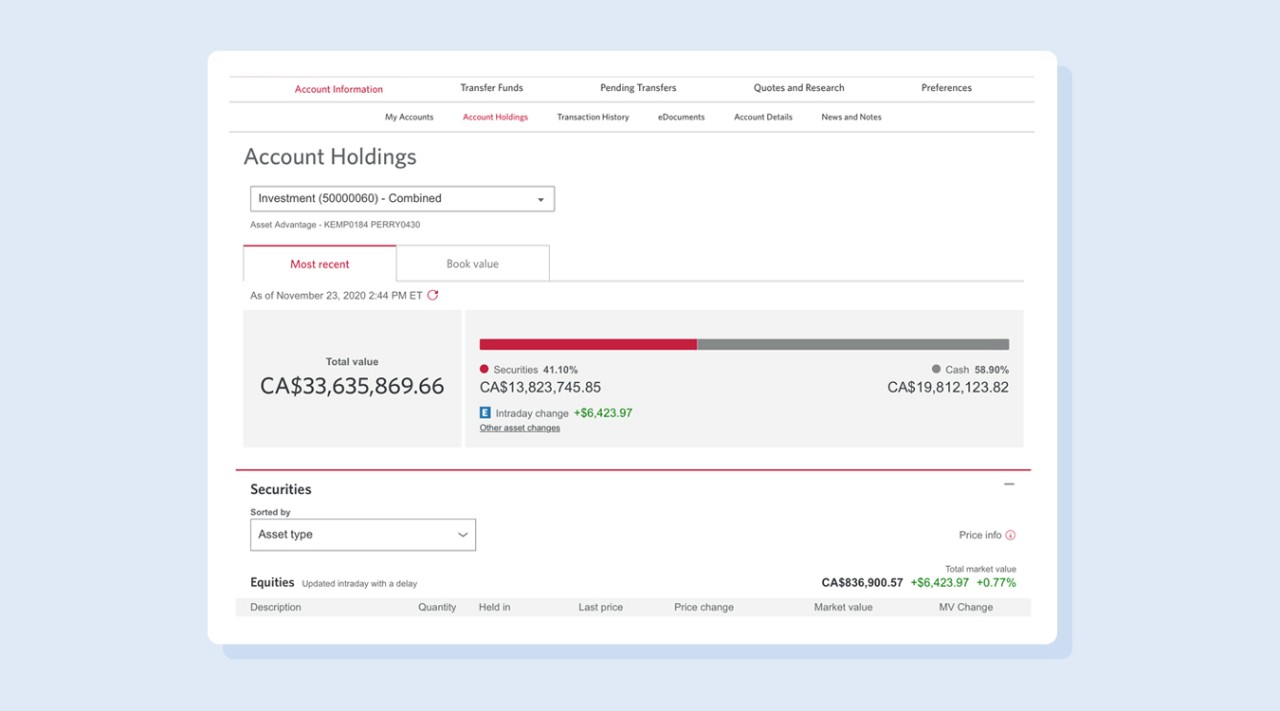Screenshot from a banking website displaying account holdings. The top navigation bar includes tabs such as "Account Info," "Transfer Funds," "Pending Transfers," "Quotes and Research," "Preferences," "My Accounts," "Account Holdings," "Transaction History," "E-Documents," "Account Details," and "News and Notes." The "Account Holdings" tab is highlighted in red, indicating the current page.

The page shows the "Most Recent" view with a red banner that also reads "Most Recent." Data is updated as of November 23rd, 2022, at 4 p.m. Two options, "Most Recent" and "Book Value," are present, with "Most Recent" currently selected.

The account's total value is listed at CAD $33,635,869.66. The asset allocation includes 41% in securities like stocks, and 58.9% in cash holdings. The total market change for the day is a positive CAD $6,000, reflecting a notable increase in the account's value.